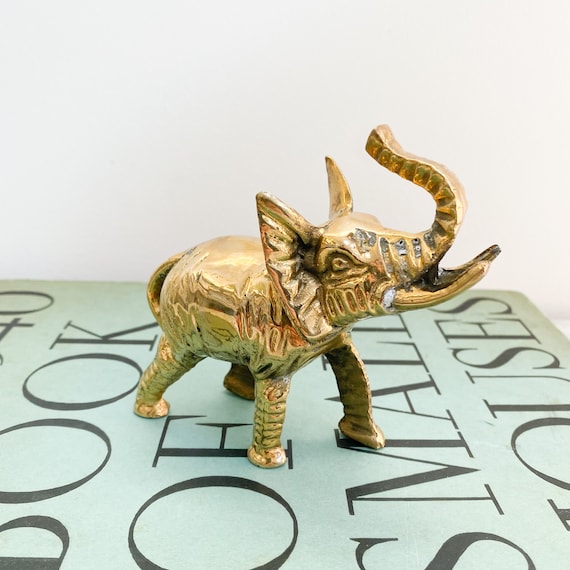This detailed photograph captures a small elephant figurine, which appears to be made of gold-colored metal, showcasing meticulous craftsmanship. The elephant is depicted standing atop a teal book, with prominent text partially readable as "Book of Small...". The background of the image is whitish, which contrasts well with the vibrant colors of the figurine and the book. The elephant is intricately detailed, with visible skin wrinkles, folds of fat on its legs, and expressive features in the eyes, ears, and trunk. The male elephant, with its gold tusks, is shown in a dynamic pose, lifting its head high and raising its trunk toward the sky, its ears erect as though bracing to charge. The positioning of its front legs, spaced wide apart, further accentuates the sense of movement and readiness in this beautifully crafted decoration.